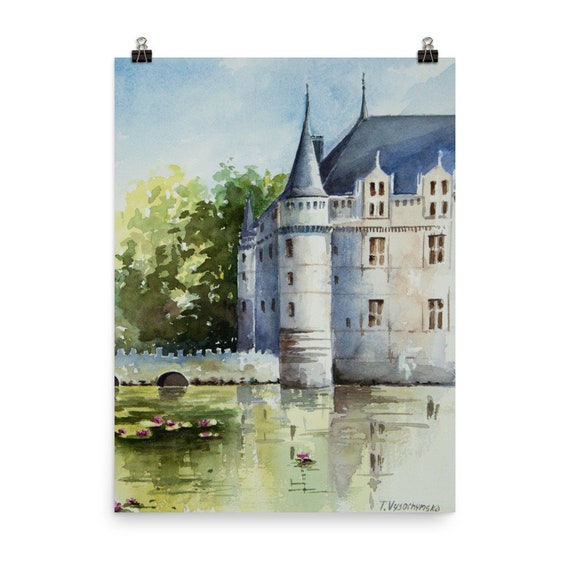This meticulously detailed watercolor painting features an old-world castle set in a serene landscape, masterfully captured in muted colors. The castle, constructed of beige and white brick with numerous small clustered windows, boasts tall towers capped with dark blue tips and a matching dark blue roof. A picturesque stone bridge extends from the castle, featuring decorative squares at its peak and an arched opening beneath, which likely allows water to flow or a gondola to pass.

In the foreground, a tranquil pond reflects the entire scene, its water shaded in olive and green hues. The pond is dotted with lily pads and adorned with delicate pink and purple flowers. To the left of the castle and the pond, tall trees rise, their colors progressively shifting from dark blue-green near the castle to lighter yellowish-green hues as they stretch towards the background.

The backdrop of this enchanting scene is a cyan blue sky, interspersed with wispy, almost translucent white clouds. The painting, held by two black clips, resides on an all-white background, with a subtle signature reading "T.V.Y.S." at the bottom right corner, indicating the artist’s mark. The entire composition exudes a sense of calm and timeless beauty, inviting the viewer into a tranquil, historic world.